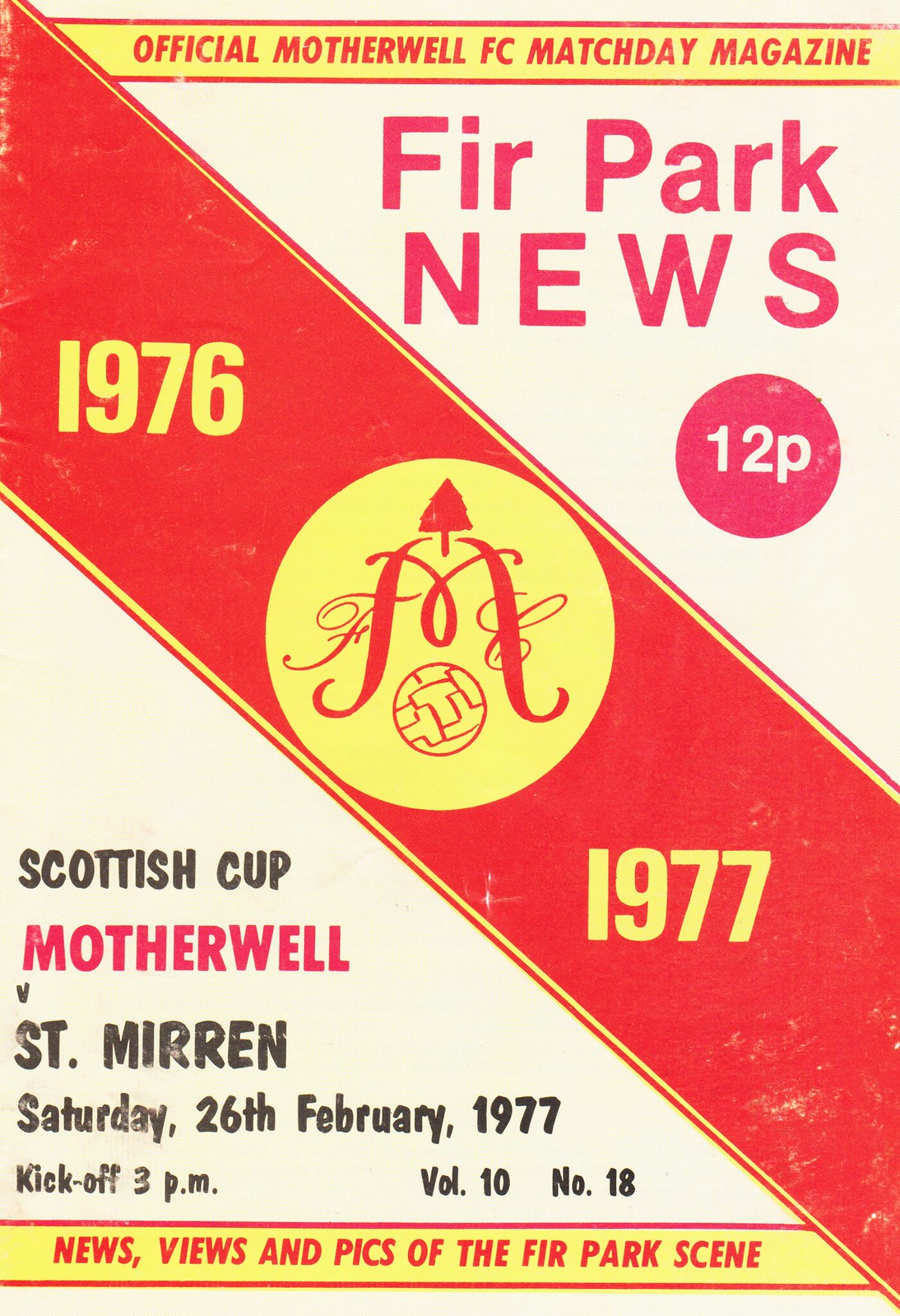This image showcases the cover of the "Official Motherwell FC Match Day Magazine" for a soccer match. The background features an off-white color resembling yellowing paper. Dominating the design is a distinct red diagonal stripe running from the top left corner to the bottom right, bisecting the cover. Centered within this stripe is a round yellow dot emblazoned with the Motherwell FC logo, featuring a stylized soccer ball beneath a tree.

At the top of the cover, the title "Official Motherwell FC Match Day Magazine" is prominently displayed in red text. Near the top, there's a red circle with "12p," indicating the magazine's price of 12 pence. Text towards the left side provides event details: "Scottish Cup Motherwell vs. St. Mirren, Saturday, 26th of February 1977, kickoff 3pm." Additional information includes "volume 10, number 18."

Towards the bottom, a horizontal yellow stripe highlights the tagline "news, views, and pics of the Fir Park scene," referencing the venue's name. The years "1976" and "1977" are printed diagonally in alignment with the stripe's direction. All these elements form a vivid and detailed portrayal of this vintage match day program cover.